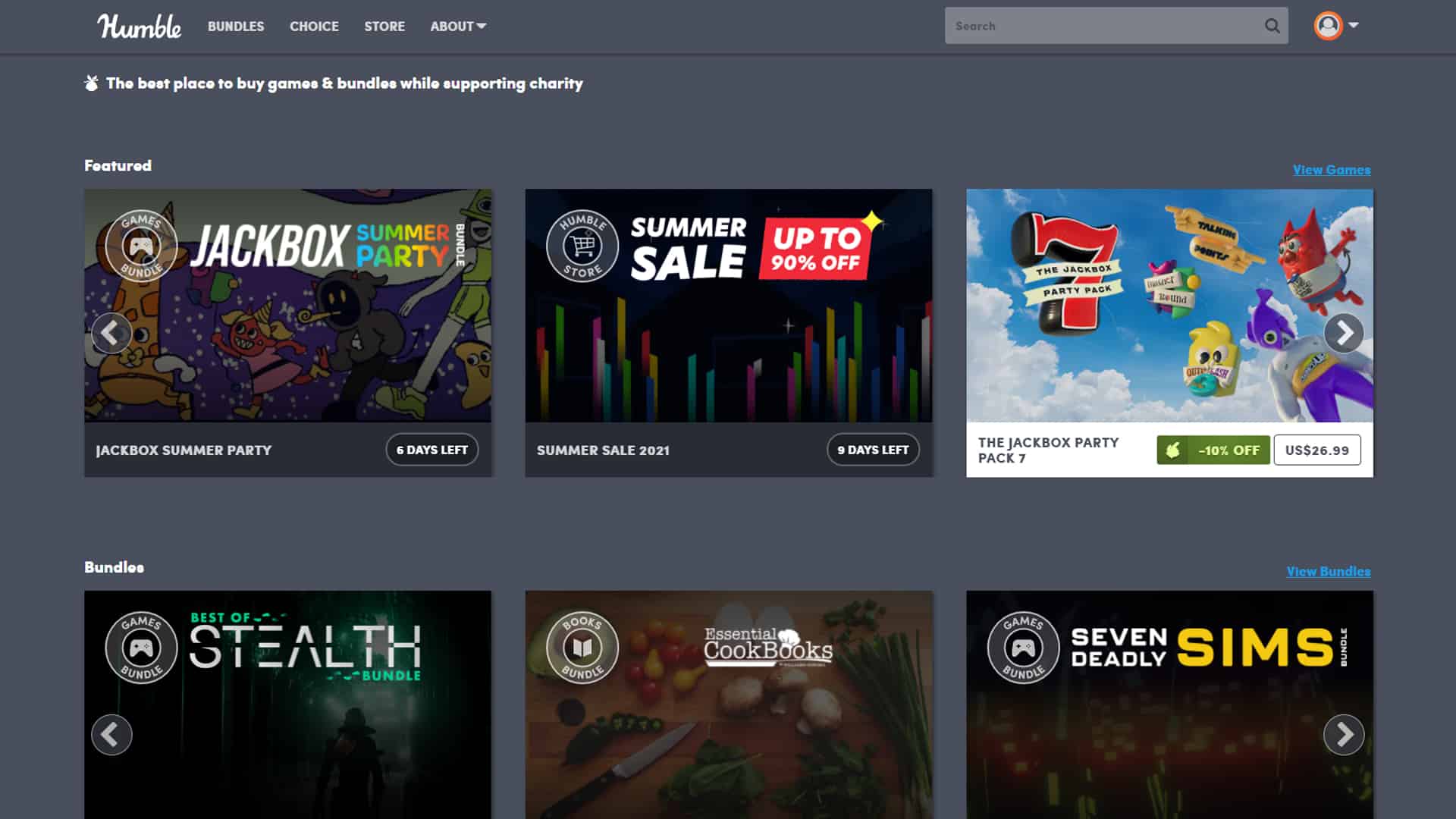This is a detailed screenshot of a website with a gray background. In the upper left corner, the word "Humble" is displayed in white, cursive letters. To the right of "Humble," the navigation bar continues with the words "Bundles," "Choice," "Store," and a drop-down menu labeled "About." Further right, there is a search field and a profile drop-down menu. Beneath the navigation bar, a slogan reads: "The best place to buy games and bundles while supporting charity." 

Below the slogan, there are two rows of images, each containing three boxes that appear to feature video games or promotions. In the first row, the leftmost box is titled "Jackbox Summer Party," the middle box advertises a "Summer Sale up to 90% off," and the rightmost box features a red "7" with text indicating "The Jackbox Party Pack." 

The second row is labeled "Bundles" and highlights different themes: the leftmost box says "Stealth," the middle box says "Cookbooks," and the rightmost box says "Seven Deadly Sims."